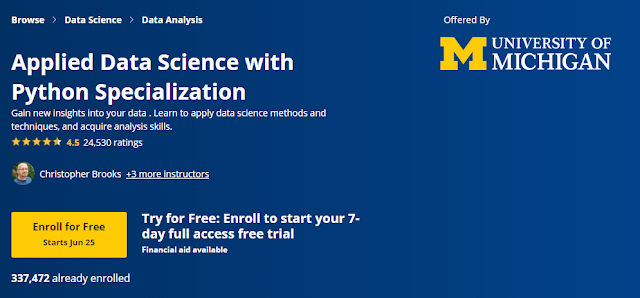The image displays a web page for the University of Michigan's "Applied Data Science with Python Specialization." The primary design element is a large blue square with prominent white text. In the top left corner, the words "Browse, Data Science, and Data Analysis" are displayed in white. On the top right corner, the text "Offered by the University of Michigan" is highlighted in bold white lettering.

Inside the blue square, the course title "Applied Data Science with Python Specialization" is prominently noted, followed by a brief description detailing the course's benefits. It highlights the opportunity to gain new insights into data, learn to apply various data science methods and techniques, and develop comprehensive analysis skills. The course has received significant feedback, with 24,530 ratings averaging 4.5 stars.

At the bottom of the blue square, there is a smaller yellow square indicating that you can enroll for free, with the course starting on June 25th. Additional notes include options to try for free with a 7-day full access trial and the availability of financial aid. It is also mentioned that 337,472 people have already enrolled in the course.